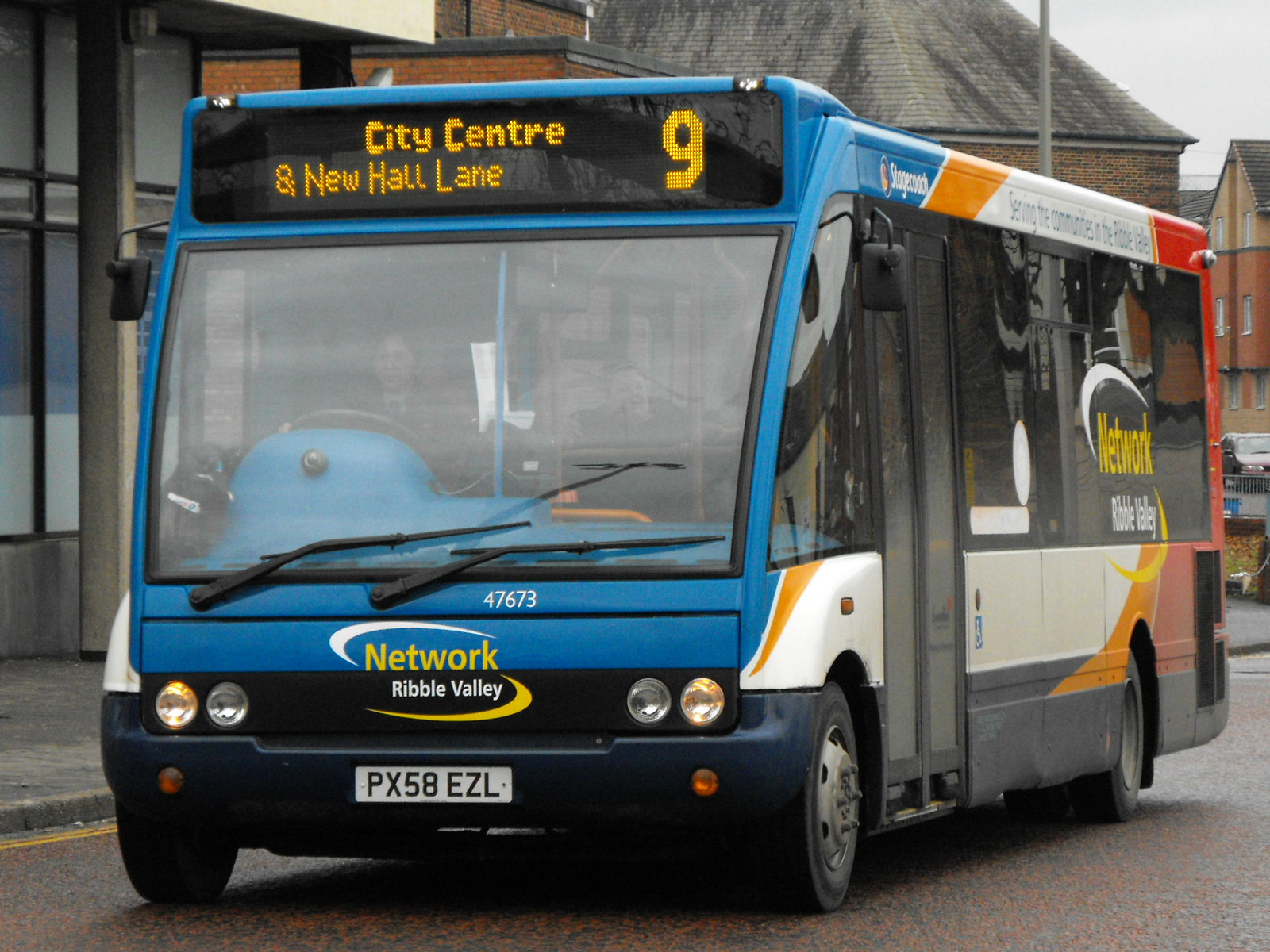The image is a detailed color photograph of a single-decker bus, captured in landscape orientation from street level. The bus is prominently positioned, driving towards the left side of the frame. Its front features a large, cubic shape with a broad windscreen, and the main color at the front is blue. Above the windscreen, a digital display reads, "City Centre & Newhall Lane" in orange dots, alongside the number "9" on the right side. 

The vehicle's license plate, PX58 EZL, is situated at the bottom, under which the text "Network Ribble Valley" is presented in yellow, flanked by semicircular plate-like designs. The bus also features a logo with concentric swirls in yellow and white on the front. 

On the side of the bus, which is adorned with orange, white, red, and blue stripes, the text "Network Ribble Valley" is visible on the windows. The top corner of the bus bears the inscription "Stagecoach," alongside blue text that reads, "serving the commuter in the Ribble Valley." For security, a camera is mounted on the back top corner of the bus, above several vents. 

The road beneath the bus is paved in black and orange, with double yellow lines marking the sides. The scene includes background details of buildings and town settings indicating an outdoor, urban environment. Visible through the bus's large windows are the driver holding a black steering wheel and a few passengers.